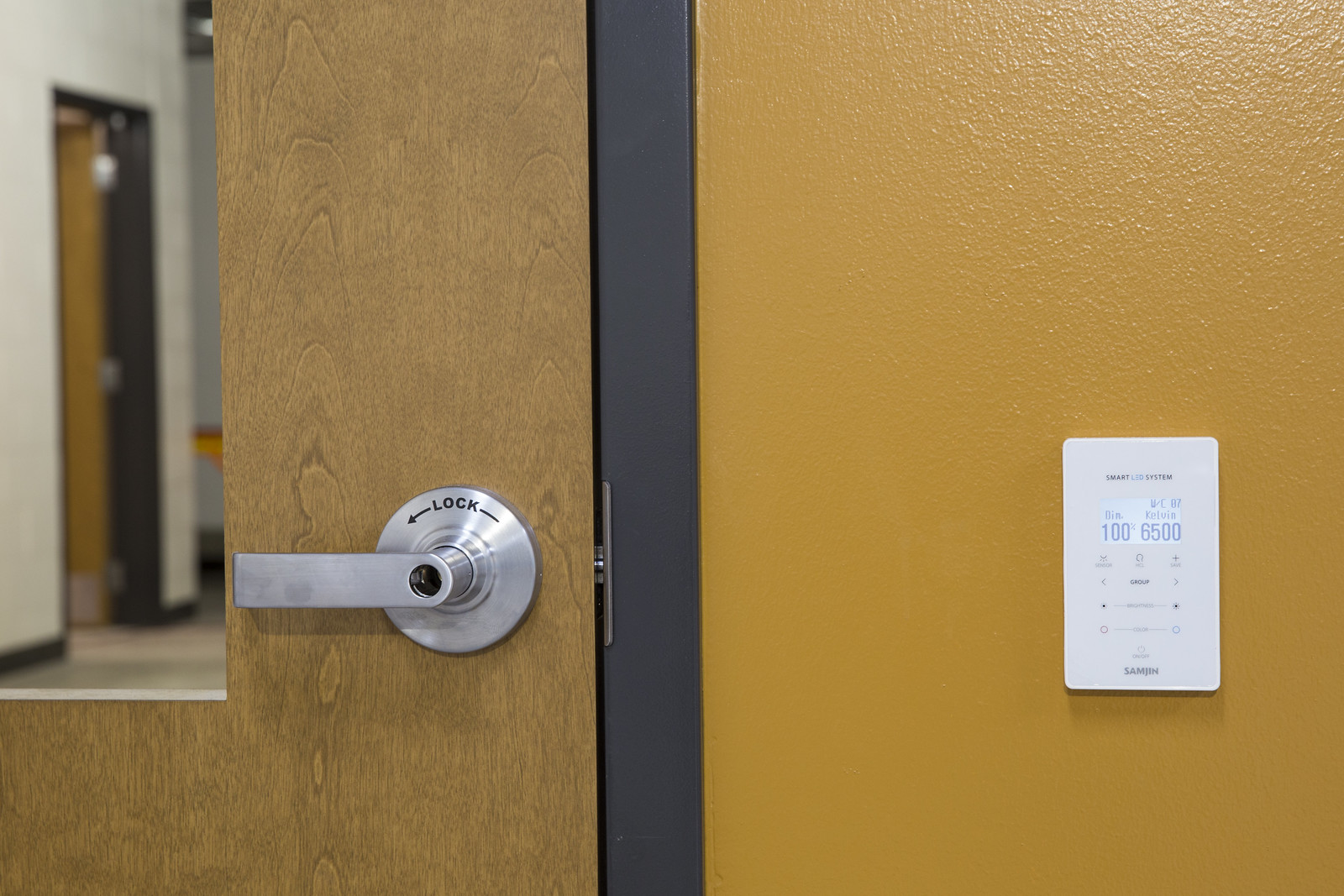This photograph evokes a sense of warmth and humidity, possibly due to the wet mustard-colored wall with its glossy and textured surface. The wall holds a sign reading, "Smart LED System," detailing specifications such as "DIN 100%, Kelvin 6500," with sections for "Group" navigated by arrows indicating direction, as well as "Brightness" and "Color." At the bottom of the sign, the brand "Samjin" is mentioned in bold letters.

Adjacent to this vibrant wall is a black metal door frame, supporting a wooden door with a solitary pane of glass. The door features a stainless steel handle, accompanied by a sign with the word "Lock" and an arrow pointing left, suggesting that pulling the handle down would secure the door. The setting appears to be within an educational institution, such as a high school or college, inferred by the presence of an identical door visible in the hallway beyond.